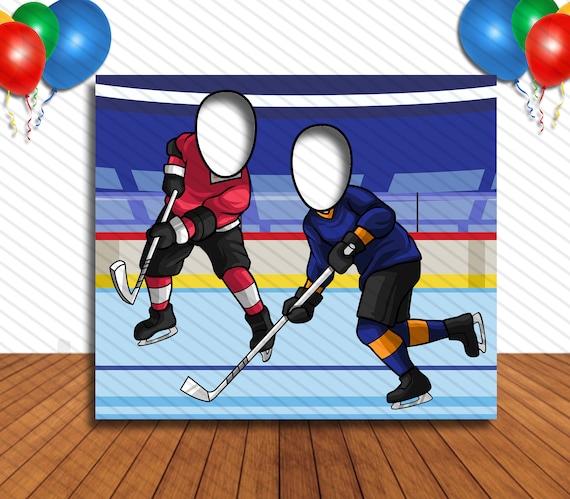The image is an illustration designed for interactive fun, likely intended for a kid's party. It depicts two ice hockey players front and center, each with cut-out ovals for faces where people can put their own faces through to pose for photos. The player on the left is dressed in a red jersey, black shorts, red stockings, black gloves, and black ice skates, while the player on the right is in a dark blue jersey, black shorts, blue stockings, black gloves, and black ice skates. Both are holding gray hockey sticks and appear to be in action poses. The scene is set against a white background with a brown hardwood floor beneath the signage. The top corners of the image feature colorful balloons in blue, green, yellow, and red. Additionally, light gray diagonal lines run across the background from the upper right to the lower left. The setting seems to mimic an ice rink with empty stands visible in the distance.